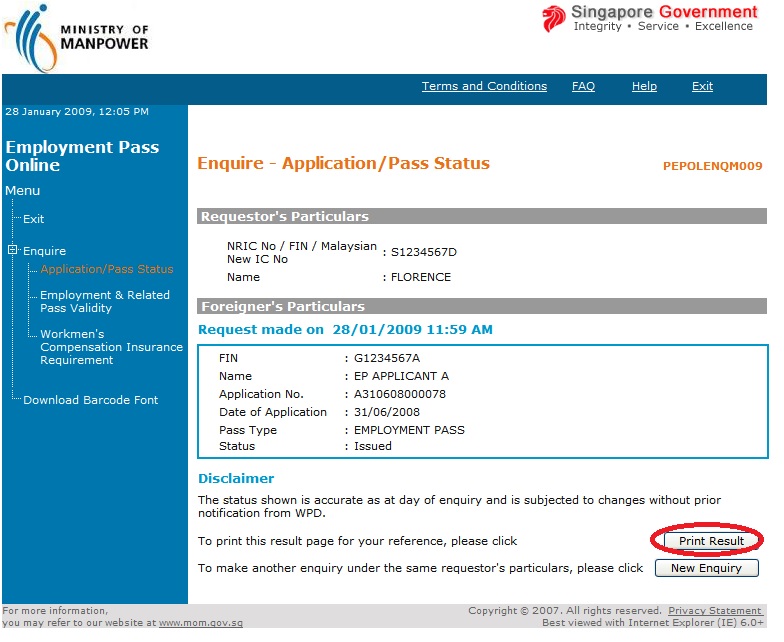The image features a webpage with a white background, representing the Ministry of Manpower, Singapore Government. In red text, it displays key attributes such as "Integrity," "Service," "Excellence," along with navigation options including "Terms and Conditions," "FAQ," "Help," and "Exit." The timestamp is noted as 28 January 2009, 12:05 p.m. 

The content is centered around an "Inquire Application Pass Status" section, specifically for "People in QM009." It categorizes data under "Requesters' Particulars" and lists details like "NRIC/FIN/Malaysian New ICNO," with an individual named Florence.

Also, under "Owners' Particulars," details include a request made on 28 January 2009 at 11:59 a.m., displaying a number with letters and numbers inside a blue rectangle for the FIN. The document states the name as "EP Applicant A," followed by an application number with an 'A' prefix, and notes the application date as 31 June 2008. The "Pass Type" is listed as "Employment Pass" with the status marked as "Issued."

Furthermore, the page includes a disclaimer section labeled as "Information" and features a "Print Result" button highlighted within a circle.